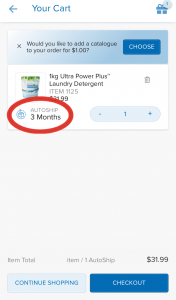In this blurry image, we see a screenshot, which appears to be taken from a shopping app on a phone. The resolution is notably low, making details somewhat unclear. At the top left corner, there is a back button pointing left, and next to it, the words "Your Cart" with each word capitalized. On the right side of the screen, there is an icon resembling a gift box with a notification badge displaying the number one.

Below this, a banner message asks, "Would you like to add a catalog to your order for $1?" with a dismissible "X" button next to it and a blue button labeled "Choose," indicating it might be an advertisement or upsell prompt.

Further down, there's an item listed: "1kg Ultra Power Plus Laundry Detergent, item 1125," priced at $31.99. The accompanying image of the detergent is predominantly white, green, and blue. To the right of this image, a red circle highlights the "Auto Ship every 3 months" option.

At the bottom of the screen, a summary states, "Item total: item 1, Auto Ship: $31.99." Below this, two buttons are available: a blue button labeled "Checkout" and a white button labeled "Continue Shopping."